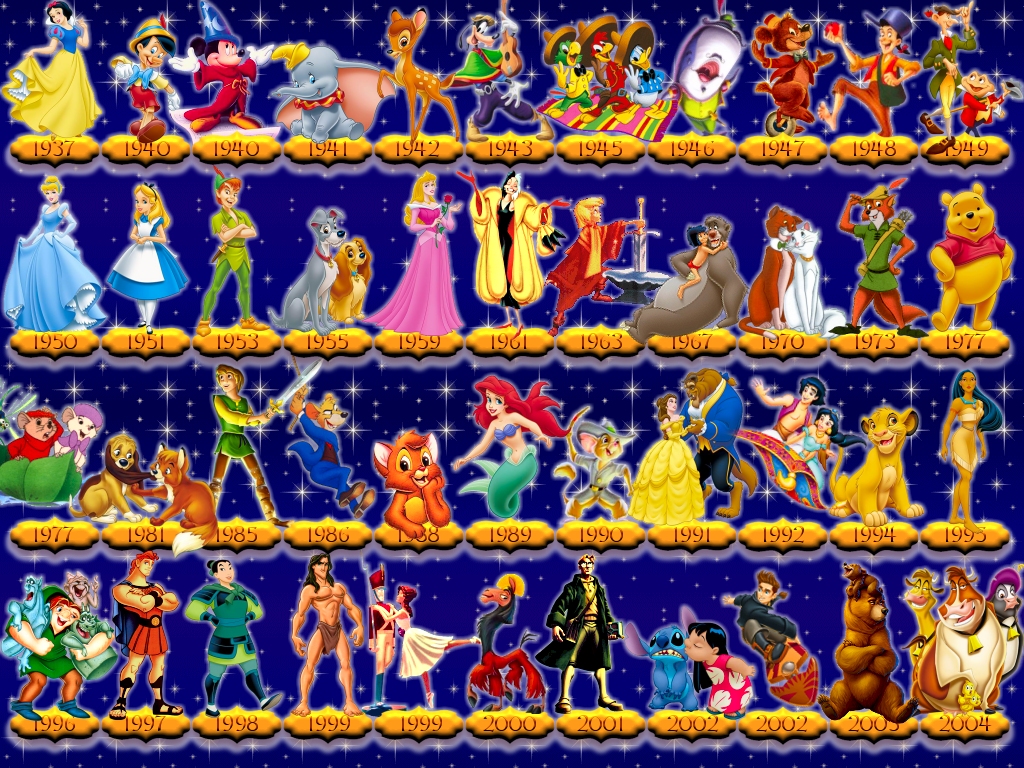This detailed poster showcases a rich timeline of Disney characters from 1937 to 2004, set against a dark blue, starry night sky. Each character is colorfully detailed, outlined with a bluish glow, and accompanied by a year-banner in gold with the release year inscribed in a darker gold shade. The poster features 44 individual images organized in four rows and eleven columns. Starting with Snow White from 1937 at the top left, it includes iconic characters such as Pinocchio, Mickey Mouse, Dumbo, Bambi, Goofy, Donald Duck, Winnie the Pooh, Simba from The Lion King, Beauty and the Beast, Ariel, and Peter Pan. The timeline culminates in 2004 with lesser-known characters that resemble cows and other small animals. The background is adorned with a variety of stars, adding to the magical Disney ambiance.